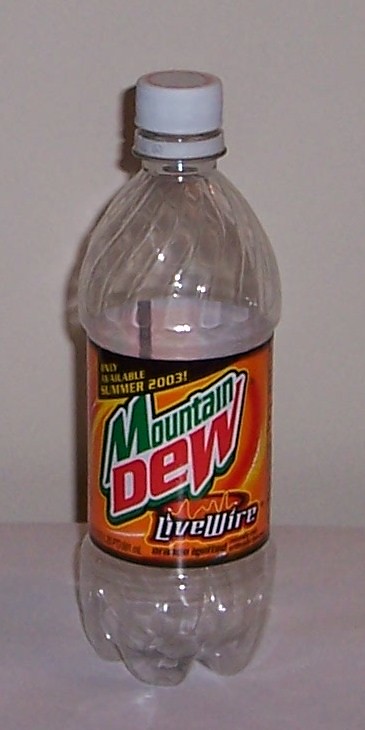This close-up photograph depicts an empty Mountain Dew Live Wire bottle, positioned on an off-white surface against an off-white wall. The bottle is made of clear plastic, featuring molded swirl designs at both the top and bottom for added texture. Its cap is white with red writing on it, and it shows signs of having been opened, as the two plastic pieces of the cap have separated. 

The label, wrapped around the center of the bottle, predominantly showcases an eye-catching blend of dark orange, tangerine, and yellow hues. The Mountain Dew logo, with "Mountain" in green and "Dew" in red, stands out prominently. Underneath the logo, "Live Wire" is displayed in white text outlined in black, against an orange background adorned with brighter orange lines and a heartbeat-like squiggly line above the text. The label also features a distinctive black triangle protruding downward from the top. For added stability, the bottle's base includes four indentations to help it stand upright.